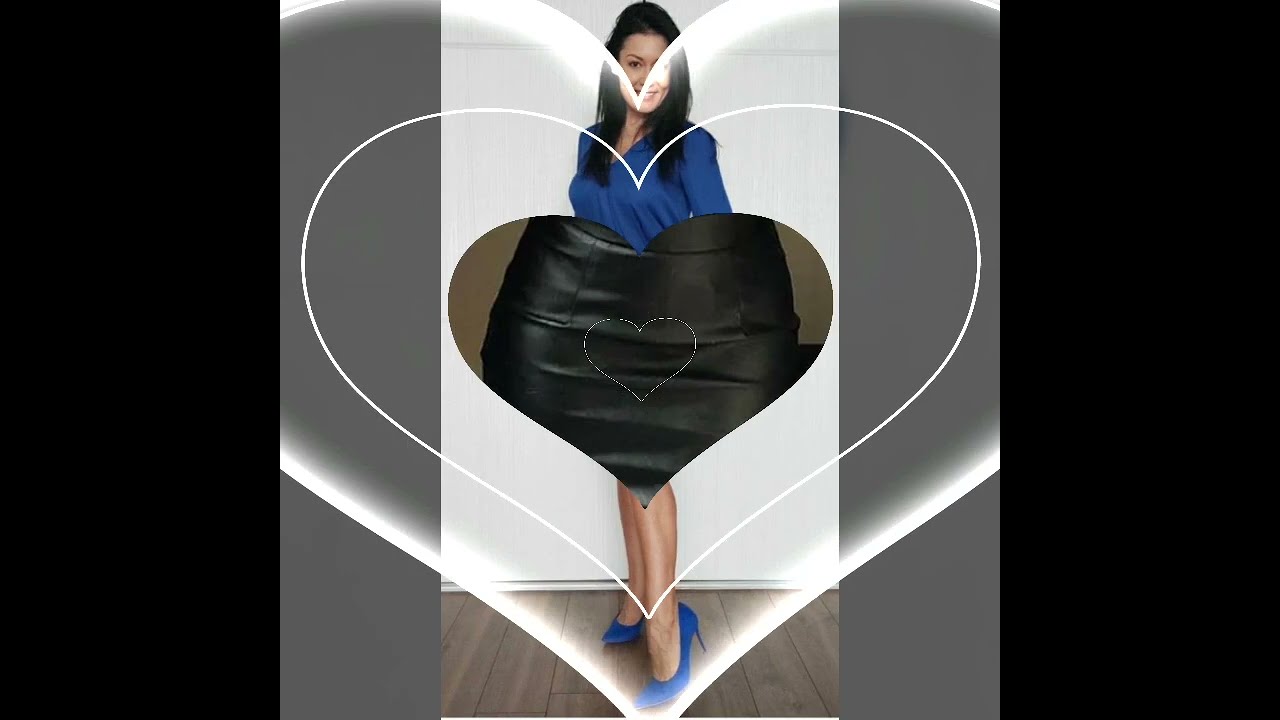The image showcases a young woman with dark black hair, smiling, and dressed in a blue blouse paired with a leather skirt and matching blue high heels. She stands on dark brown wooden floorboards against a plain white wall. The key element of the image is the leather skirt, particularly accentuated by graphic art—four white, see-through hearts surround her, including a smaller heart prominently displayed on her skirt which draws attention to it. The composition and graphic elements suggest the image is intended for advertising the leather skirt, emphasizing its style and desirability.